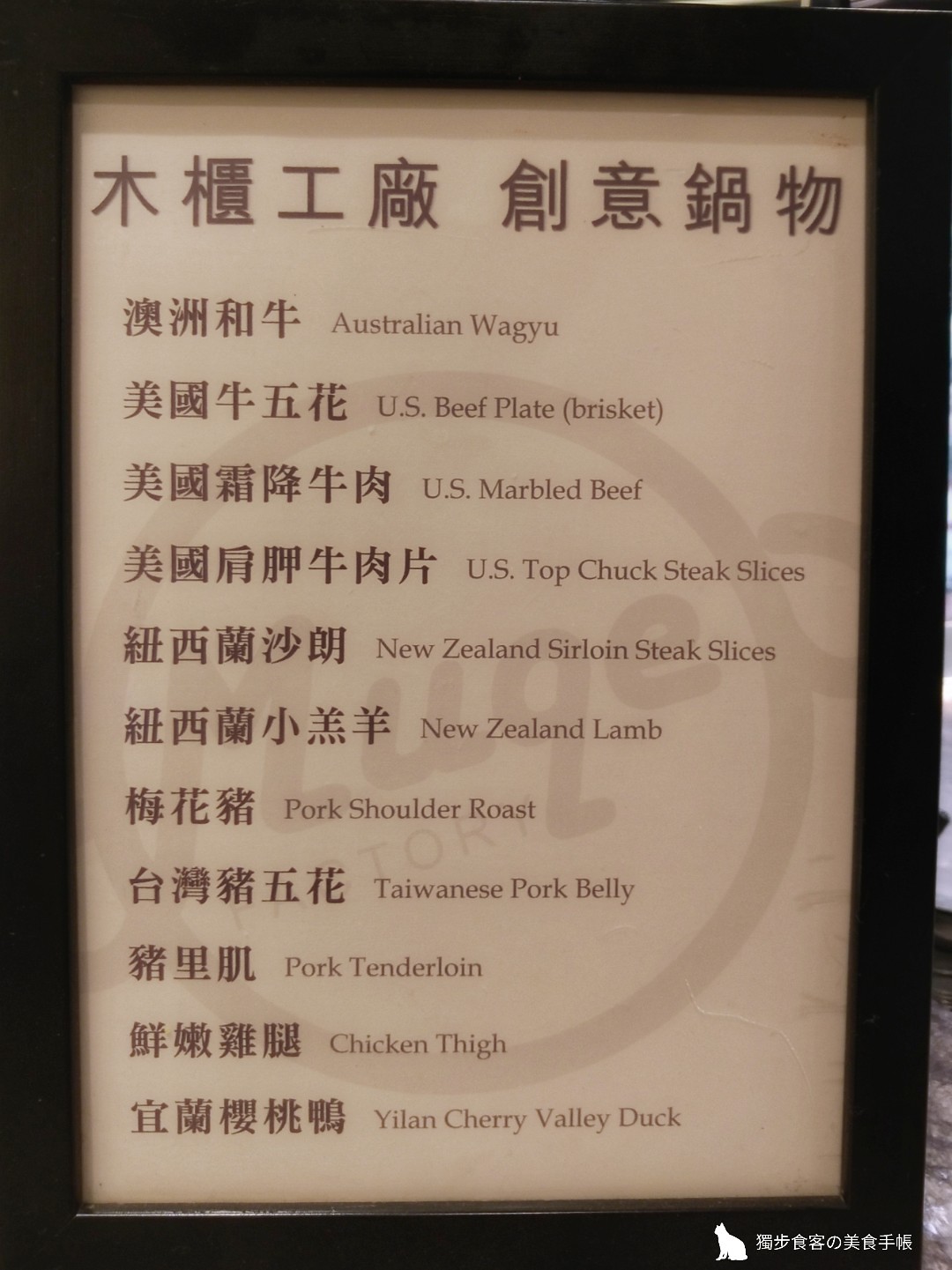The image showcases a framed menu, predominantly in what appears to be pinyin, the Romanization system for Chinese characters. The menu is printed on light tan-colored paper with a subtle, large white circle watermark featuring the restaurant's logo or name, "Muge to." The text is in a darker brown shade, contrasting elegantly with the paper's light background.

At the top of the menu, the pinyin characters are displayed. The listed items include:

1. **Australian Wagyu** - Written in English, with corresponding pinyin characters.
2. **US Beef Plate Brisket** - Accompanied by pinyin characters and noted as "US marbled beef" in parentheses.
3. **US Top Chuck Steak Slices** - Followed by the pinyin representation.
4. **New Zealand Sirloin Steak Slices** - Alongside its pinyin counterpart.
5. **New Zealand Lamb** - With the respective pinyin.
6. **Pork Shoulder Roast** - Rendered in pinyin.
7. **Taiwanese Pork Belly** - Listed with its pinyin translation.
8. **Pork Tenderloin** - Accompanied by pinyin.
9. **Chicken Thigh** - With its pinyin version.
10. **Yilan Cherry Valley Duck** - Presented with pinyin.

Additionally, the menu features a white silhouette of a cat, complemented by a few Chinese characters. This cat figure is positioned on what seems to be a granite countertop, providing a visually appealing element to the menu design. The overall aesthetic suggests a refined and detailed approach to presenting the diverse range of dishes offered at the establishment.